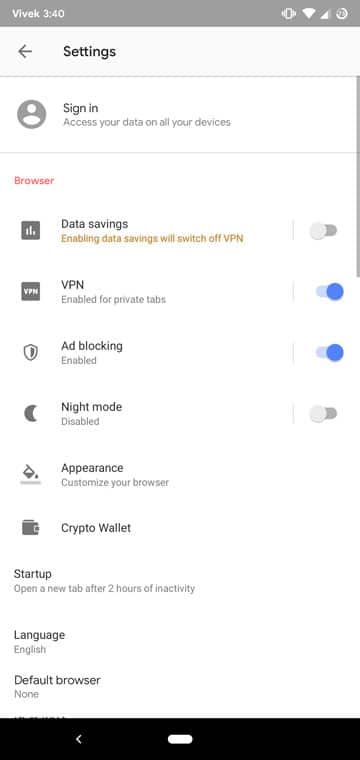In the image, we see a phone screenshot of the settings screen. At the top left, in white text, it reads "Vivec 3:40." On the top right, the Wi-Fi signal strength is fully displayed with all bars filled, and next to it, the phone signal strength shows two bars. Beside the signal strength is a vibration icon indicating the phone is set to vibrate mode.

Just below this top section, the word "Settings" is prominently displayed in black text, accompanied by a left-pointing arrow. Underneath the "Settings" title, there's a phrase instructing the user to "Sign in to access your data on all your devices." To the left of this signing prompt is a circular icon featuring a white silhouette of a torso.

Further down, we see the word "Browser" highlighted in red, followed by a vertical list of various settings options. The first item on the list is "Data Savings," followed by "VPN," "Ad Blocking," and "Night Mode." The list continues with "Appearance," "Crypto Wallet," and ends with "Startup," "Language," and "Default Browser." Under the "Language" option, the current setting of "English" is displayed.